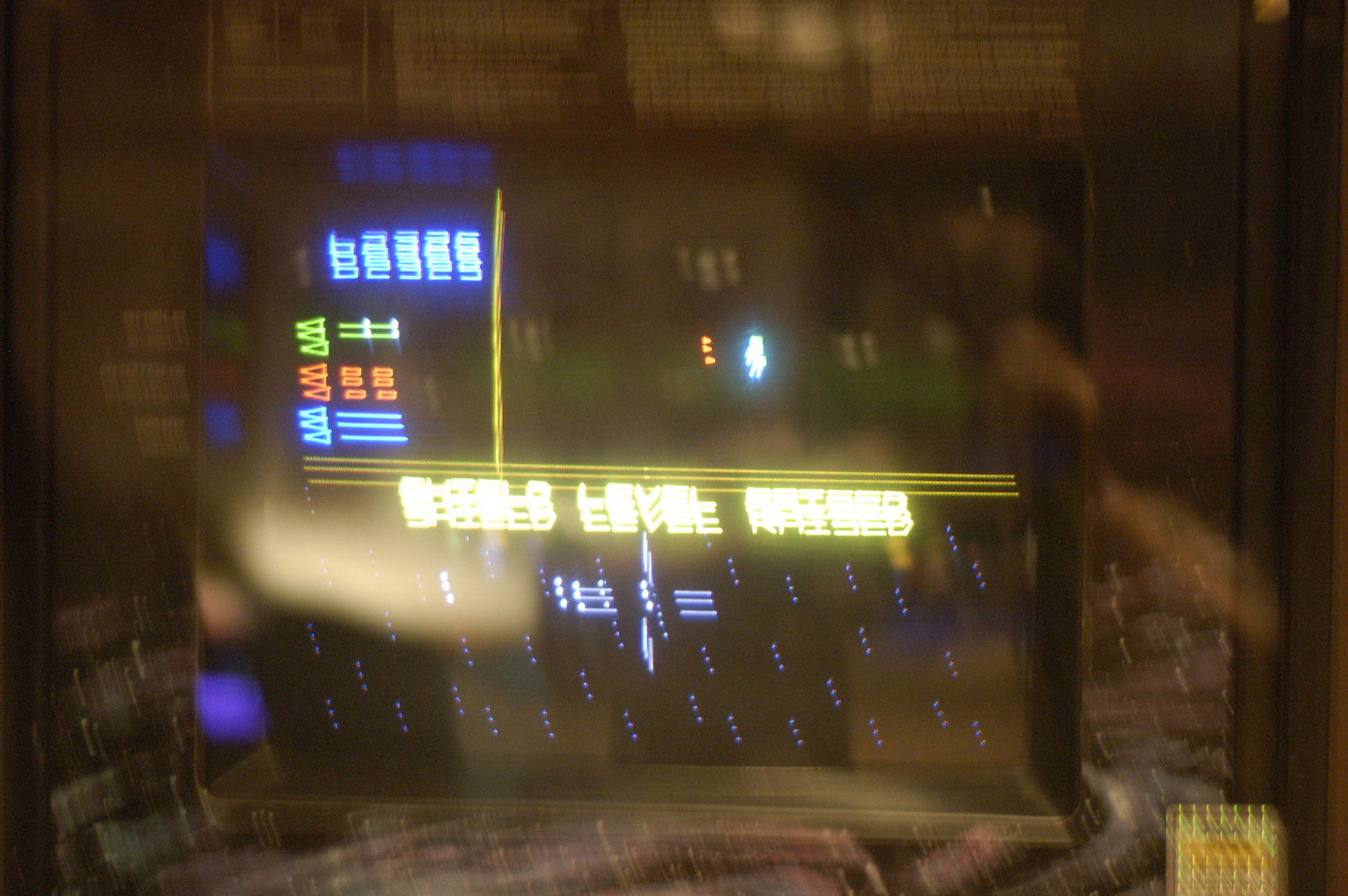This image showcases an arcade video game cabinet, prominently positioned on the left side of the image. The cabinet features vibrant side panel artwork, depicting a swirling galaxy at the bottom, encapsulating the cosmos theme of the game. At the top of the cabinet, instructions are displayed next to the screen. The photograph is taken in motion, giving the impression of a dual image overlapping slightly.

On the game's screen, the score is remarkably high, reading 62,325 at the top right corner. The game appears to be a space-themed shooter, with an image of a spaceship navigating through an outer space setting. The bottom of the screen features a target crosshair, indicating active gameplay, surrounded by stars and a shield level indicator. The shield level reads "Blue," and there are directional indicators (left, right, up, down) shown as small lines arranged in a circular configuration in the middle of the bottom section. 

A faint reflective touch can be seen on the arcade cabinet, adding a sense of depth and realism to the image. On the bottom right corner of the screen, elements of gameplay details are visible in a subtle way. Below the score on the top left of the screen, there are indicators marked in green, red, and blue, possibly representing different functions or statuses in the game. The elaborate description of the arcade cabinet and its screen details presents a captivating sight for any retro video game enthusiast.